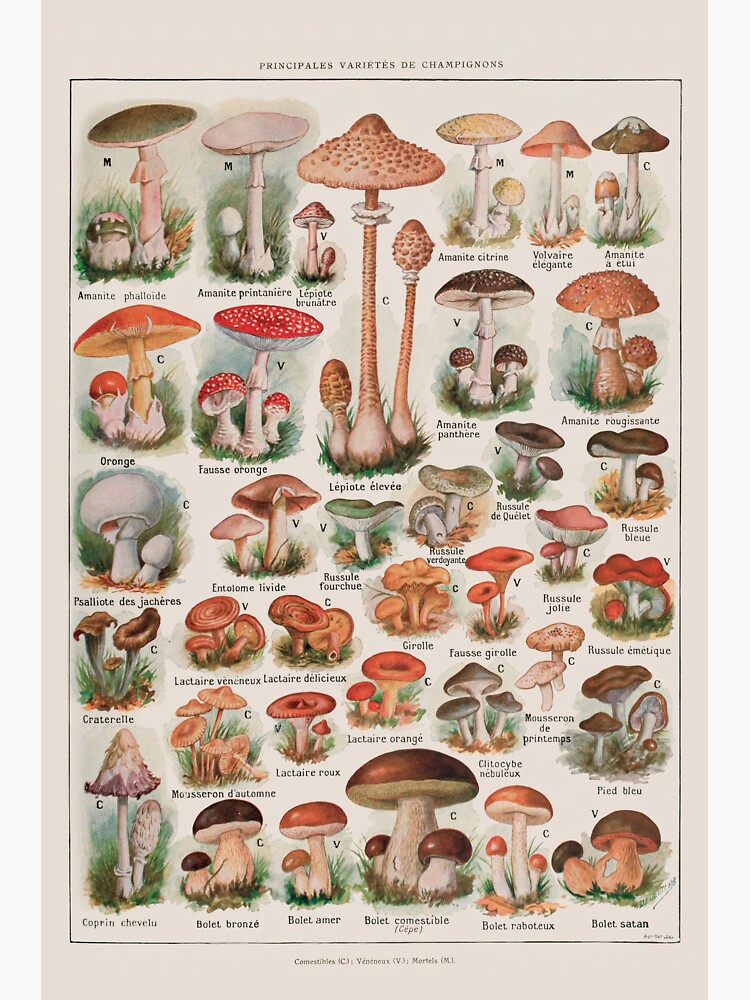The image is an illustrated poster for identifying mushrooms, titled "Principales Varietes de Champignons," which is French for "Main Varieties of Mushrooms." The poster has a thin black border framing it, with the interior depicting around 36 different mushrooms organized into approximately six rows. Each row features six or seven mushrooms of varying shapes and sizes, ranging from tall and skinny to short and squatty. The mushrooms are illustrated in an old-timey photorealistic style, showcasing red, green, and other vibrant colors. Some mushrooms are depicted with grassy or earthy backgrounds. Common mushroom shapes include toadstool with red tops and white spots, umbrella, parasol, and trumpet forms. Each mushroom has its name written below it in French, paired with a letter, often 'C' or 'V,' which might indicate the mushroom's classification or variety. Notably, the largest mushroom depicted is labeled as "Lepotes Olivo." The detailed and colorful illustrations make this poster both informative and visually engaging.